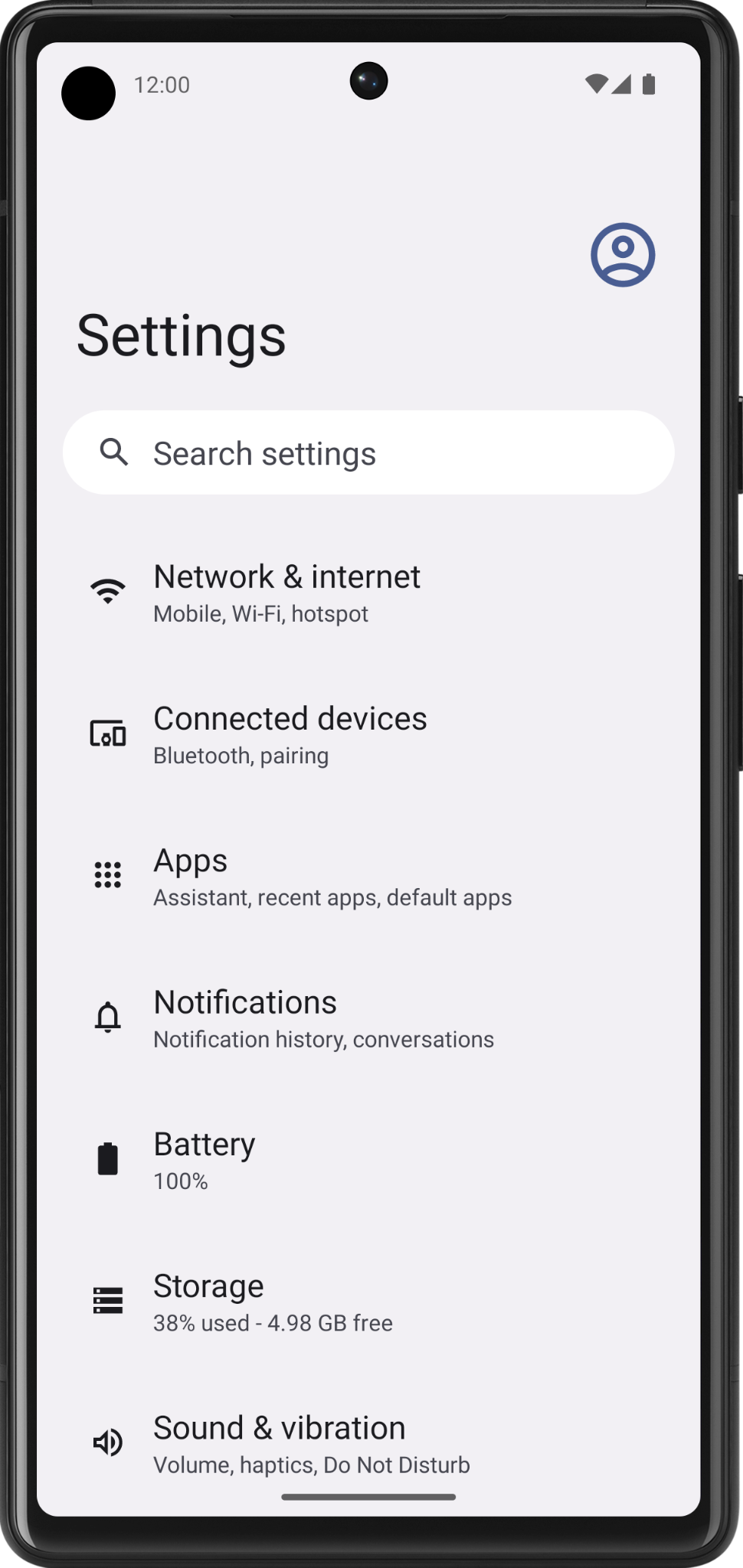The image shows a smartphone with a black outline, captured with its screen on. The phone's physical buttons are distinctly visible on the right side, including three tactile buttons. At the top left of the screen is a small circle, likely an icon or notification, followed by the time display. Centrally placed at the top is another circle, probably the front camera. The top right corner displays the Wi-Fi signal strength, network signal strength, and battery level indicator.

The primary focus of the screen is the "Settings" interface, detailed as follows:

- Directly below the battery indicator is a circular icon depicting a person's profile.
- The word "Settings" is prominently displayed in large font on the left side.
- Below it is a capsule-shaped search bar with a magnifying glass icon on the left, followed by the text "Search settings."

Descending through the options listed:

1. **Network & Internet**: Represented by a Wi-Fi signal icon, this option includes topics like mobile data and Wi-Fi hotspot.
2. **Connected Devices**: Indicated by an icon featuring a large rectangle and two smaller rectangles, covering Bluetooth and device pairing.
3. **Apps**: Marked by a grid of nine dots, this section encompasses assistant, recent apps, and default apps preferences.
4. **Notifications**: Featured with a bell icon, detailing notification history and conversations.
5. **Battery**: Displayed with a battery icon, showing 100% charge.
6. **Storage**: Illustrated by three parallel horizontal lines, indicating 38% used storage and 4.98 GB free space.
7. **Sound & Vibration**: Shown with a speaker icon, detailing volume, haptics, and do not disturb settings.

This image captures a comprehensive snapshot of the phone's settings interface, giving a clear view of each option and its corresponding icon.